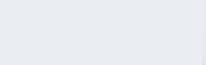The image displays a simple, light gray colored rectangle, approximately three inches in length and one inch in height. The rectangle is unadorned, lacking any internal elements, textures, or surrounding context. It appears almost as an abstract shape against a blank canvas, offering no additional details or features to describe its purpose or significance.